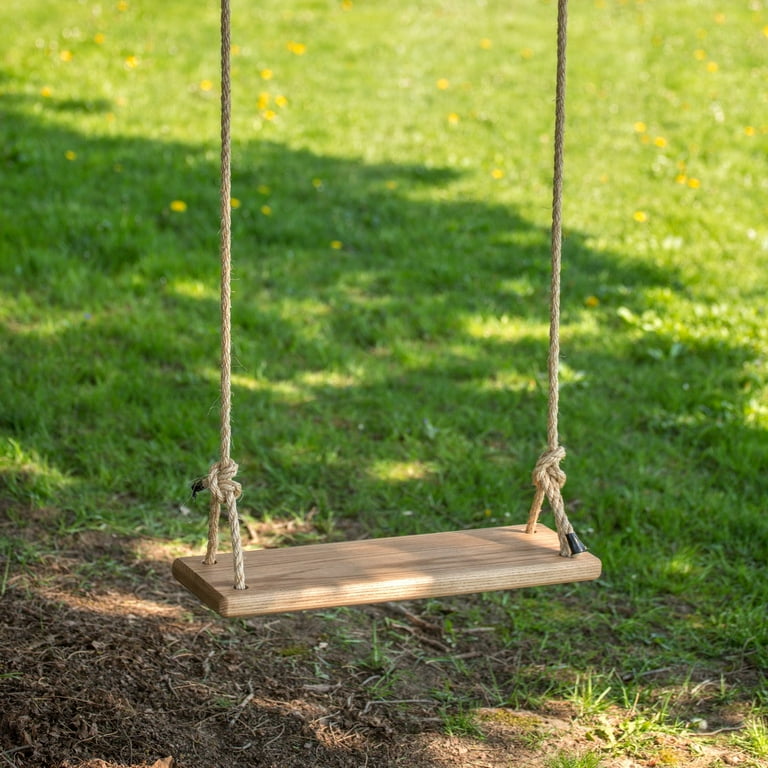The image is a detailed color photograph of a simple, yet polished wooden swing hanging from a tree. The wooden board of the swing is about 18 inches long and 8 inches wide, sanded smooth and possibly stained. It features four holes through which medium-sized tan ropes are threaded. These ropes are secured with knots just above the wood, with black tape wrapped around the ends to prevent unraveling. The swing is in the shade, casting a shadow on the ground below, which combines patches of dirt, leaves, and tree debris. The background reveals a mix of sunny and shaded grass, peppered with bright yellow dandelions, implying it's taken during the day. The image exudes a serene, outdoor ambiance with the tree's shadow stretching across the lawn, and despite its simplicity, the photograph appears professional and thoughtfully composed.